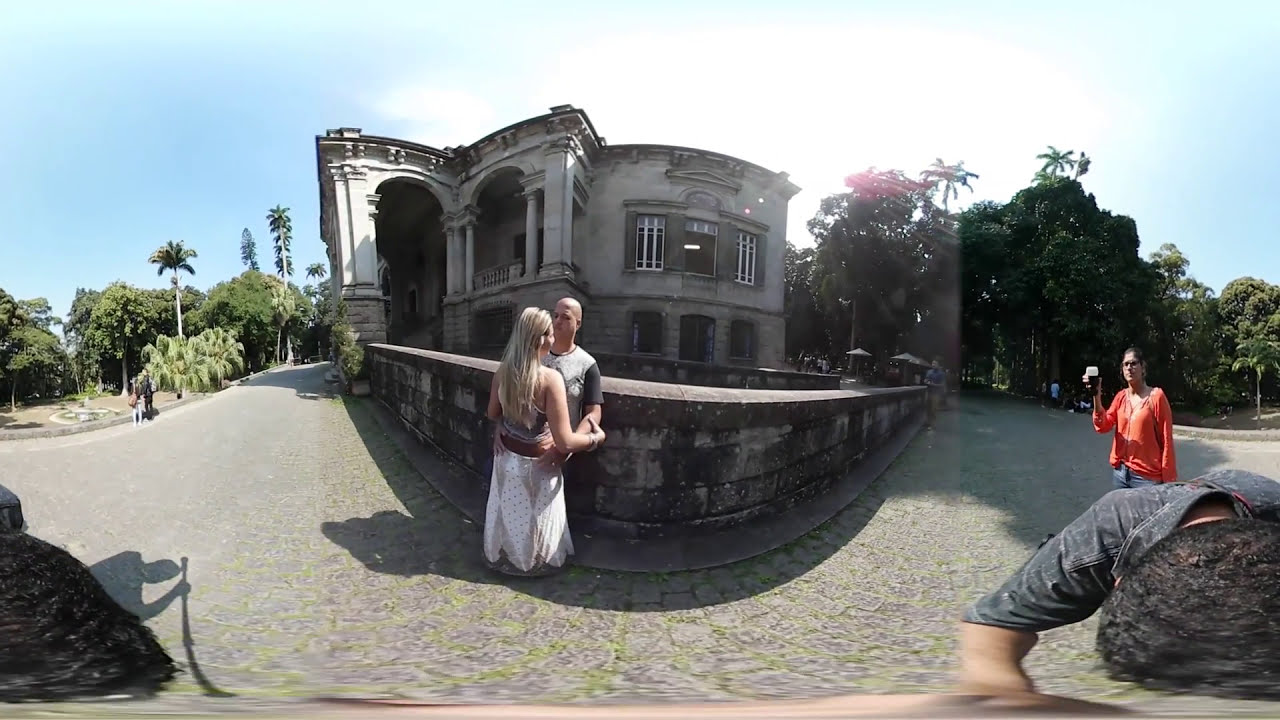The image captures a vibrant and sunny street-level panorama of a historic stone building, reminiscent of an old manor or administrative building. The scene is slightly distorted due to the fisheye effect of the panoramic shot. The building, which has at least two stories and features arched windows and doors, is framed by a circular stone wall about three to four feet high. In the foreground stands a young couple; the man has a shaved head and wears a grayish-green t-shirt, while the woman, with her long blonde hair, is clad in a white tank top and a flowing white skirt. She embraces the man, her back to the camera. To the right, a woman in an orange long-sleeve shirt captures the moment with her camera. The tropical setting is enriched with palm trees and other shady trees, as well as pink flowers blossoming on one of the trees, all under a clear blue sky. Several people mill around the historic site, emphasizing its public allure and timeless beauty.